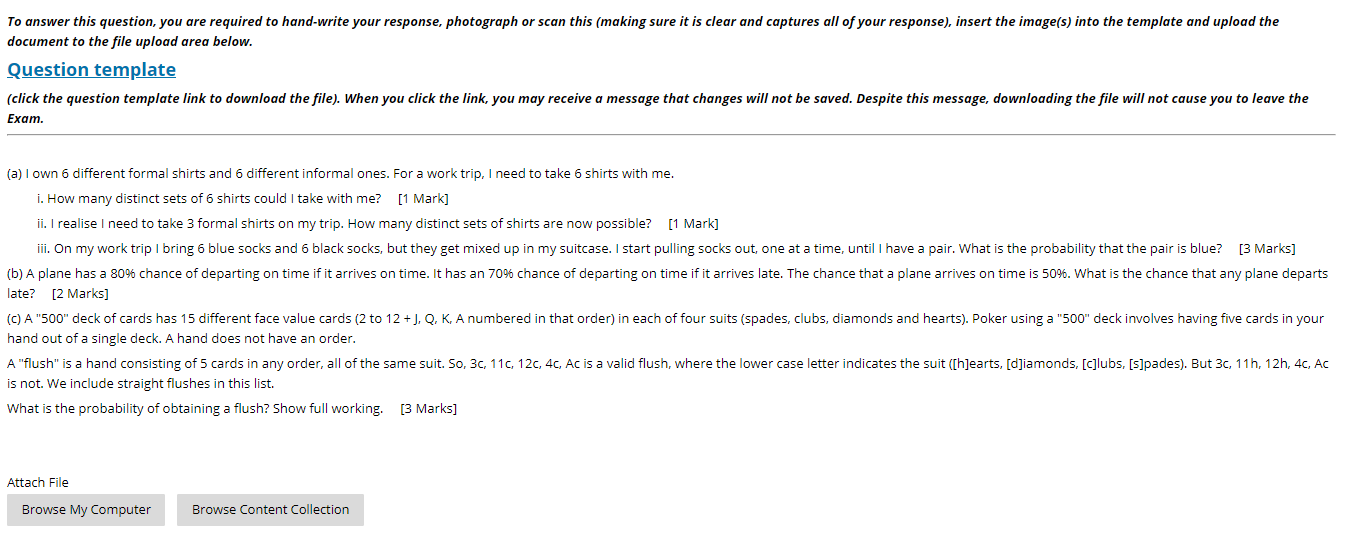The top portion of the webpage is distinguished by bold black text stating, "To answer this question, you are required to handwrite your response, photograph, and scan it. Make sure it is clear and captures all your responses. Insert the image into the template and upload the document to the file upload area below."

Below this introductory information, the webpage features a "Question Template" heading in blue, underscored by a solid line. The template is divided into several sections with different directions labeled A, B, and C.

Section A presents a scenario about shirts:
1. It states, "I own six different formal shirts and six different informal ones. For the workshop trip, I need to take six shirts with me. How many distinct sets of shirts could I take with me?" This question is marked under a sub-label "L."
2. Further, there is an additional sub-question under label "II," which reads, "I realize I need to take three formal shirts on my trip. How many distinct sets of shirts are now possible?" This part is labeled for a single mark.
3. Another question in this section states, "On my work trip, I bring six blue socks and six black socks. If they get mixed up in my suitcase and I start pulling socks out one at a time until I have a pair, what is the probability that the pair is blue?" This question is allocated three marks.

Section B delves into probability:
1. It presents the following scenario: "A plane has a 80% chance of departing on time if it arrives on time, and a 70% chance of departing on time if it arrives late. The chance that the plane arrives on time is 50%. What is the probability that any plane departs late?" This question carries two marks.

Section C includes an additional set of questions with varying marks, but the print is too small to provide further specifics.

At the bottom of the page, it instructs the user to attach files, featuring two gray rectangles labeled "Browse My Computer" and "Browse Content Collection" in bold black text.